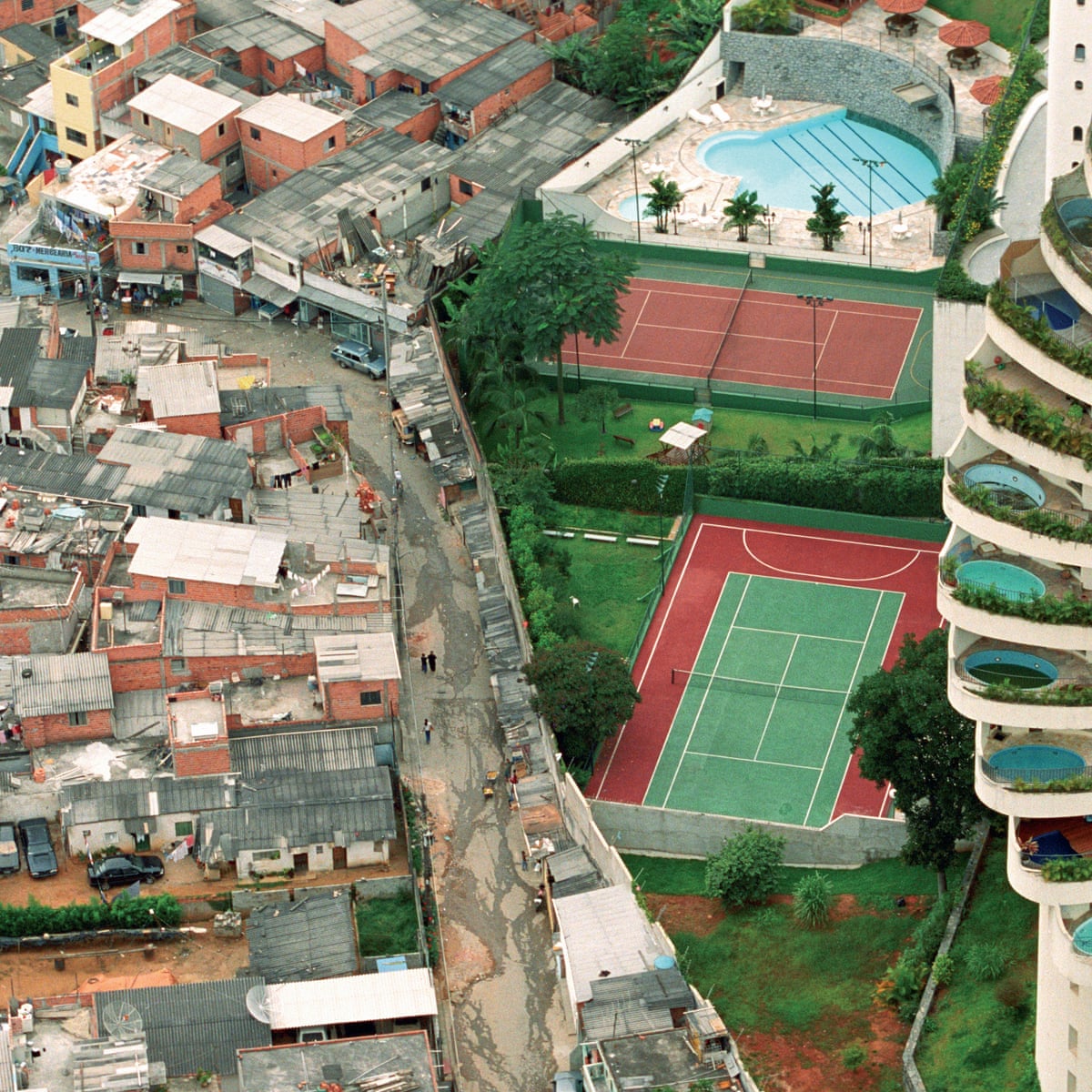An aerial photograph of a city, square in shape, captures a striking socioeconomic contrast. Dominating the center from top to bottom is a large concrete wall dividing two distinct areas. On the left, a slum-like neighborhood is evident, featuring older buildings with flat rooftops in shades of white and gray, depicting poor living conditions. Conversely, the right side showcases affluence with two tennis courts, lush green areas, and a luxurious high-rise building with multiple balconies, each sporting its own private swimming pool. The tennis courts are arranged perpendicular to each other, one with green courts and a red border, and the other with a red central court and green border. Adjacent to the courts, a round-shaped swimming pool with stone surroundings, beach umbrellas, and a stone sidewalk exude a resort-like ambiance. The scene on the right also includes beautifully landscaped greenery and decorative potted plants on balconies, further emphasizing the disparity between the wealthy area and the impoverished slum on the left.